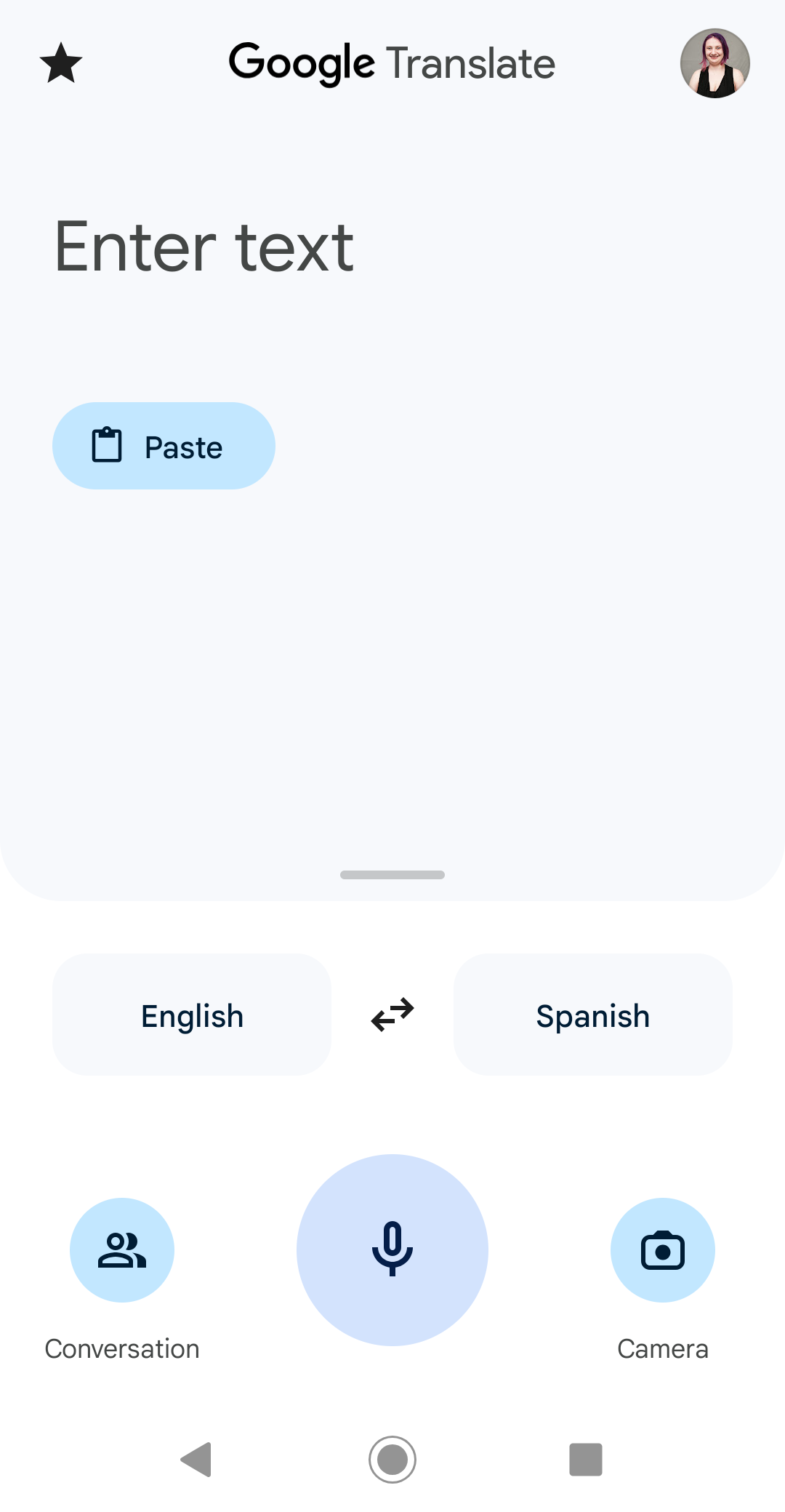This is a detailed screenshot captured from the Google Translate app interface, illustrating various interactive elements and options available for the user. In the top right-hand corner, a logged-in user profile is indicated by a small circular display picture of a woman, replacing the usual account icon. A black star is prominently placed in the top left-hand corner.

The screenshot shows that no text has been input into the translation field yet, and an icon for pasting copied text is visible, suggesting that the user may have text copied from another source ready to be translated. The language setup indicates that the translation direction is set from English to Spanish, with an easily recognizable microphone icon positioned centrally on the screen, allowing users to input spoken words for translation.

At the bottom right-hand corner, a small camera icon is present, suggesting the option to use the app's visual translation feature by capturing text via the device's camera. In the bottom left-hand corner, there is an icon featuring multiple people together, labeled "Conversation," hinting at the functionality for real-time bilingual communication.

Although no text has been input for translation yet, potential actions include pasting copied text, using the microphone for voice input, or accessing the camera for visual translation.